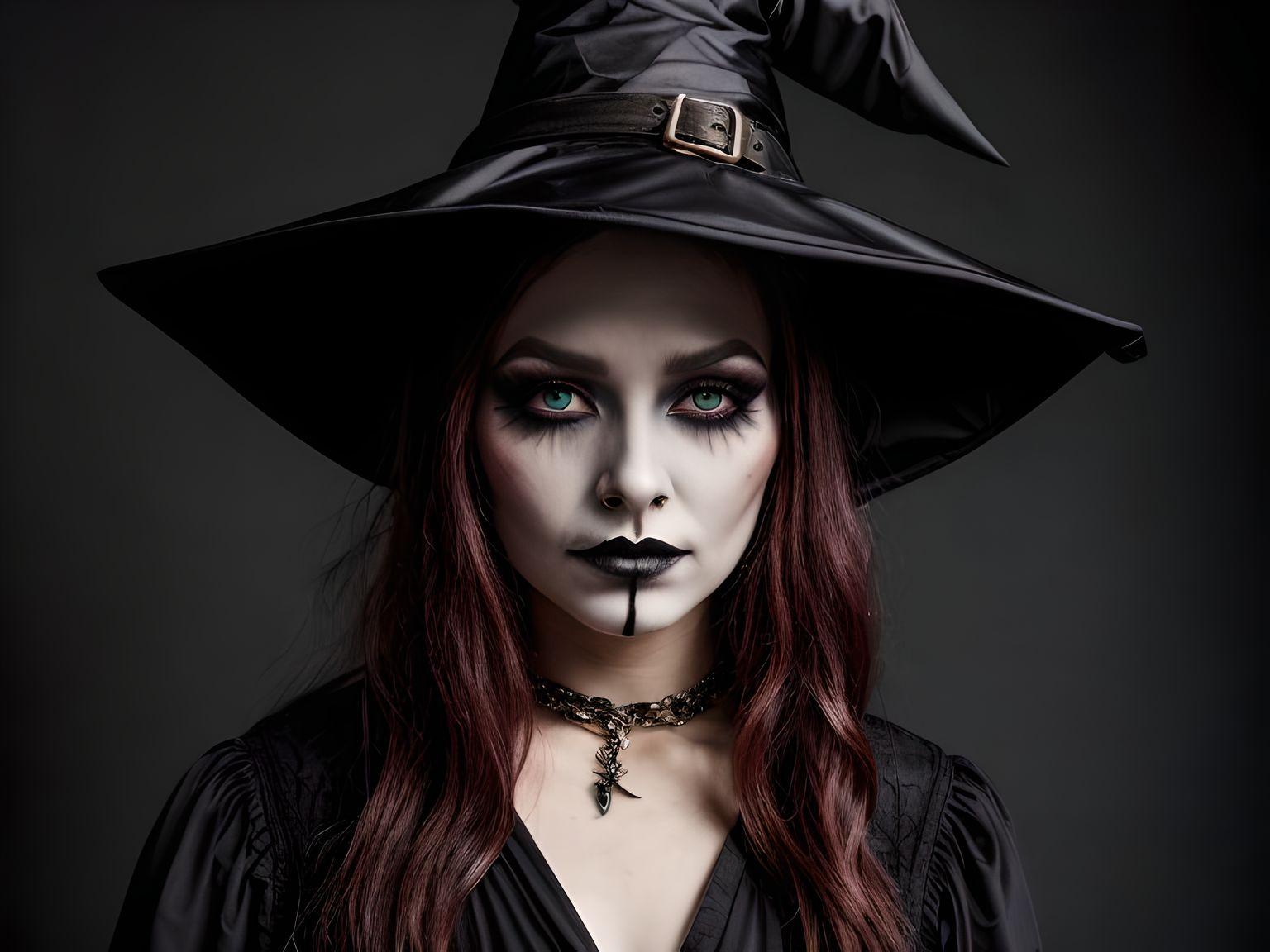This AI-generated portrait captures a woman dressed as a witch, set against a dark charcoal, gradient background. Her appearance is meticulous, almost too perfect, hinting at its digital creation. She wears a shiny, broad-brimmed witch hat with a slightly drooping pointed top, accentuated by a belt buckle. Her face is strikingly pale, painted white, with heavy black eyeshadow framing her thick, arched eyebrows and prolonged mascara, giving her a dramatic 'spider leg' eyelash effect. Her piercing, bright green eyes are vividly unsettling, with asymmetric pupils encroaching onto the waterline. A bold black lipstick adorns her lips, from which a black line extends down to her chin, enhancing her eerie aura. Her dark burgundy hair falls in soft waves just past her shoulders. She is dressed in a witchy gown featuring a deep V-neckline with loose, puffy sleeves, and accessorized with a metal choker resembling a chain, potentially with a snake emblem. This detailed ensemble, coupled with the impeccable editing, and the crispness of the portrait, underscores the sophisticated, synthetic nature of the image.